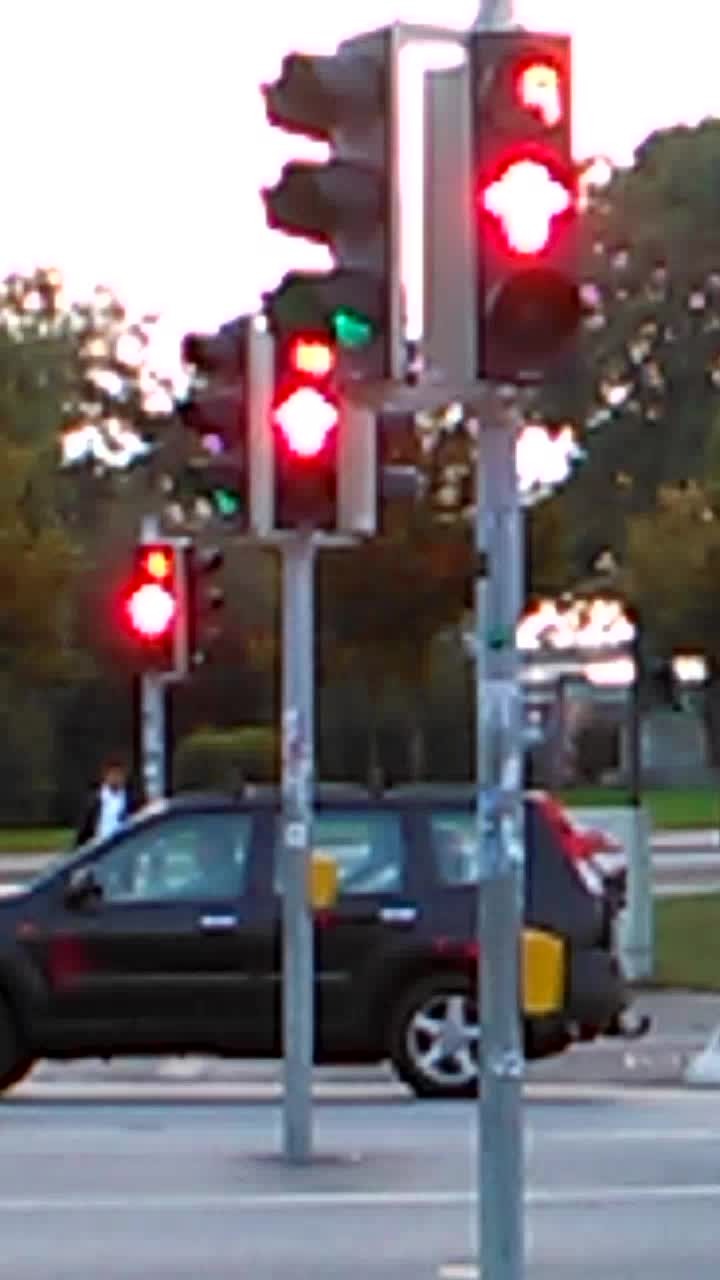This grainy, vertically framed photograph captures a urban street scene with a distinct late evening or early morning ambiance. At the forefront, a dark-colored SUV, either black or dark blue, is stationary, likely at a red light, as three traffic lights in sequential order all display a red signal. The vehicle, slightly blurred, has a visible driver, though indistinguishable in gender. Positioned behind the SUV, a pedestrian appears to be waiting to cross the road. The scene is lined with a gray paved road, marked by a white dividing line, and bordered by lush trees in the background, suggesting a nearby park or woodland area. The overall low resolution and the specific angle of a setting or rising sun give the photograph a compelling and atmospheric quality.